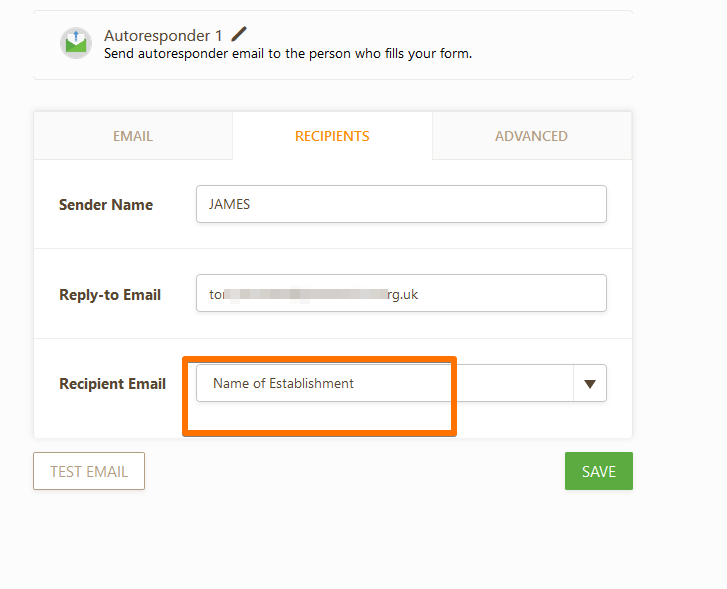This image is a cropped screenshot from a section of a website's settings page dedicated to configuring an autoresponder. At the top of the section, the title "Autoresponder 1" is displayed, accompanied by a pencil icon for editing the title. Directly below this, there is an instruction that reads, "Send autoresponder email to the person who fills your form."

The main body of the section is divided into three categories: "Email," "Recipients," and "Advanced." Below these categories are fields labeled "Sender Name," "Reply To Email," and "Recipient Email." Next to "Sender Name" and "Reply To Email," there are text boxes where information can be entered. The "Recipient Email" field features a drop-down box, which currently shows the "Name of Establishment" and is highlighted in red, indicating an error or required action.

In the bottom left corner of this section is a button labeled "Test Email," which is currently grayed out and inactive. On the bottom right, there is a green "Save" button. The entire background of the settings page is gray, while the background within the main configuration box is white, providing a clear visual distinction between different areas of the page.